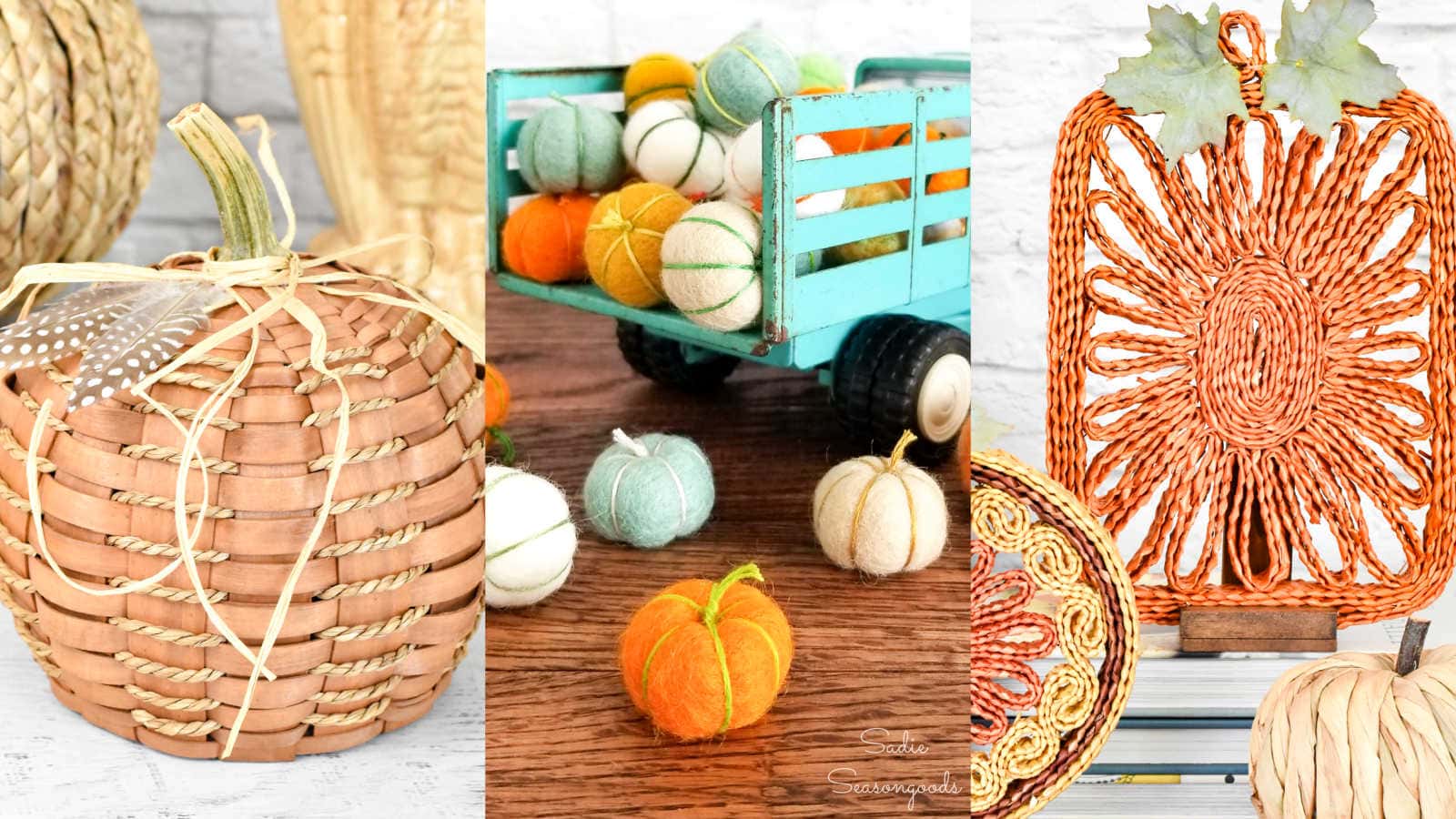This detailed collage, reminiscent of an autumn-themed interior design magazine spread, comprises three vertically divided images, all harmonizing to capture the essence of fall decor. On the left, a beige and tan woven pumpkin, intricate in its basket weave texture with a green stem and accented by wrapped brown string, stands as a rustic centerpiece. The middle image features the back half of a light blue toy truck, artfully laden with a charming assortment of stuffed and felt pumpkins in a spectrum of autumn hues, including white, orange, light blue, and dark orange. This scene is set against a wooden table, enhancing its festive appeal. The right side showcases a burnt orange woven trivet, characterized by a central flower design within its rectangular frame, and adorned by green maple leaves at the top, adding a complementary touch to a white raffia pumpkin set at the bottom. This carefully composed collage encapsulates the warmth and rich textures of fall decorations.